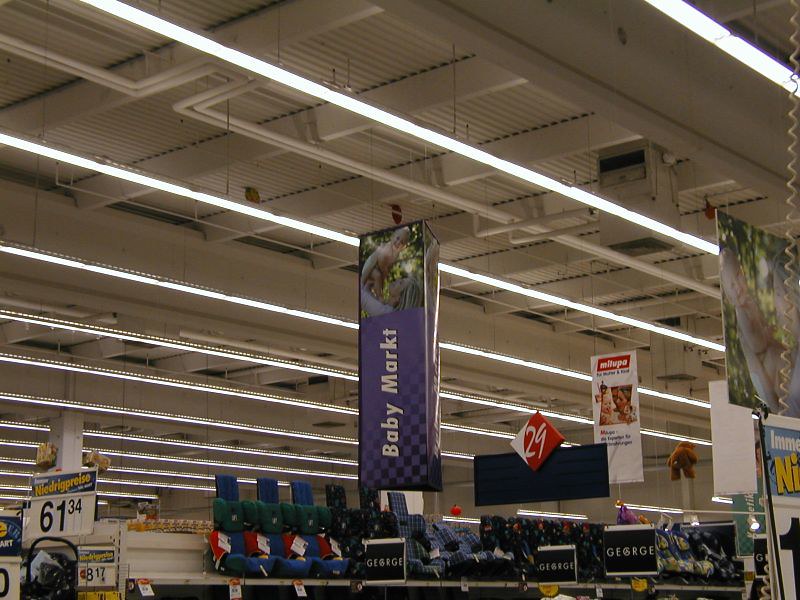This photograph captures a detailed view of a baby products section within a retail store. At the center of the image, a prominent sign hangs from the ceiling, featuring a photograph of an infant against a backdrop of black, blue, and white. The sign reads "Baby MARKT" in white font. Surrounding the sign, several baby car seats are displayed, with some sporting green hues and others adorned with blue and white stripes. Additional signage and an aisle marker are also visible; the aisle marker has a navy base with the number "29" displayed above it in bold red and white. Fluorescent lighting illuminates the scene, and the overhead industrial-style ceiling is white and adds to the utilitarian aesthetic of the store.